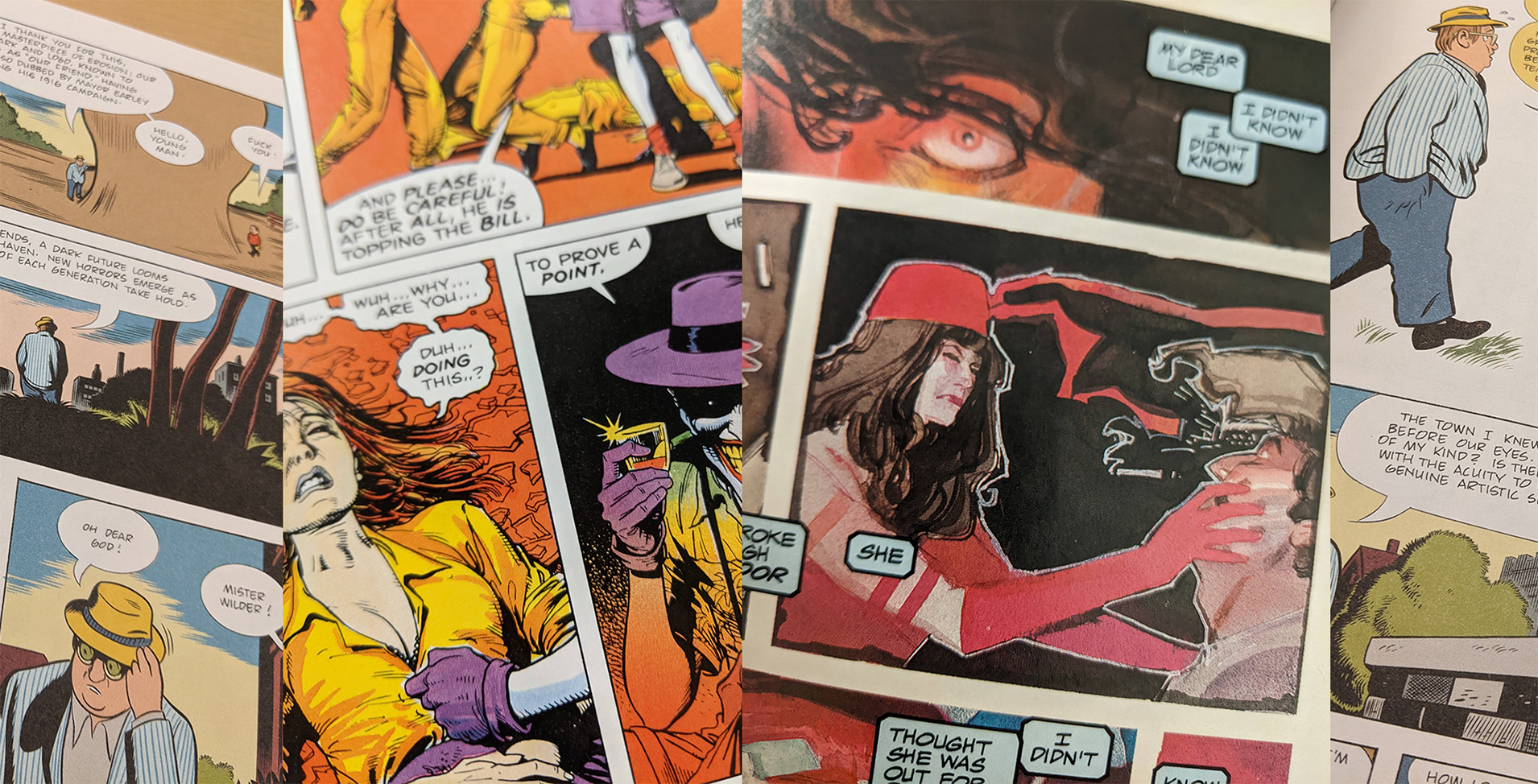This is a vivid collage of colorful comic panels arranged vertically. On the far left, the focal point is a man who seems to be a detective, dressed in a blue pinstriped sport coat, a white button-up shirt, and a yellow-brimmed hat. The background features various desert flora, like cacti, suggesting he is walking through a desert environment. This character reappears on the far right, now in a close-up shot, wearing the same distinct blue pinstriped blazer and yellow hat, looking to his right.

The second strip from the left features a notorious character resembling the Joker from Batman, engaging in some mischief. Moving to the third strip, a woman wearing long red gloves and a red hat with flowing brown hair is visibly angry as she grabs a man’s face. Her gloved hand covers his mouth, signaling an intense interaction.

In the far-right comic panel, above the reappearing detective, a rotund man looks off to his right. Below him is a snippet of text, and further down, a tree and a building are illustrated. Adjacent to these panels, a woman lies on the grass unzipping her yellow jacket, revealing a hint of her cleavage. Next to her, the Joker-like figure is captured in the act of taking her photograph, adding to the chaotic and engrossing narrative spread across these dynamic panels.